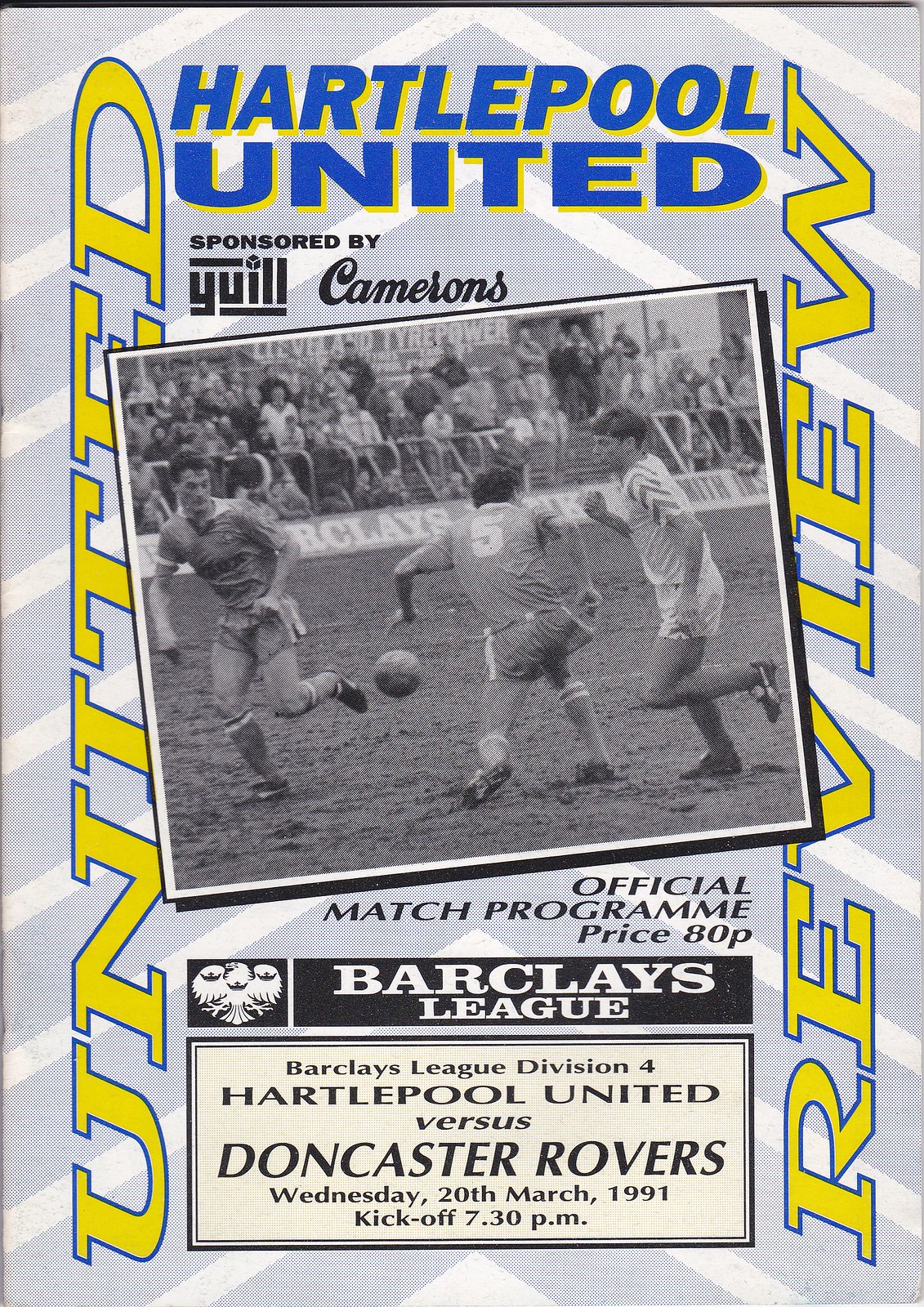The image is a color cover of an official match program for a soccer game, featuring a gray and white background with blue and gold lettering. Dominating the center of the cover is a slightly tilted black and white photograph of three young men or older boys in soccer uniforms actively engaged in a match, with a soccer ball in mid-air between them. The background of this dynamic shot includes spectators in the stands.

At the top in blue lettering, it reads, "Hartlepool United sponsored by YUILL and Cameron's." The central photograph is encased in a square frame. Below it, the text details crucial information about the event: "Official Match Program, Price 80p, Barclays League, Barclays League Division IV, Hartlepool United vs. Doncaster Rovers, Wednesday, 20th March 1991, Kickoff 7.30pm." On the left side of the cover, the word "United" is written vertically in bright yellow letters, and on the right side, the word "Review" is also written vertically in the same bright yellow font.